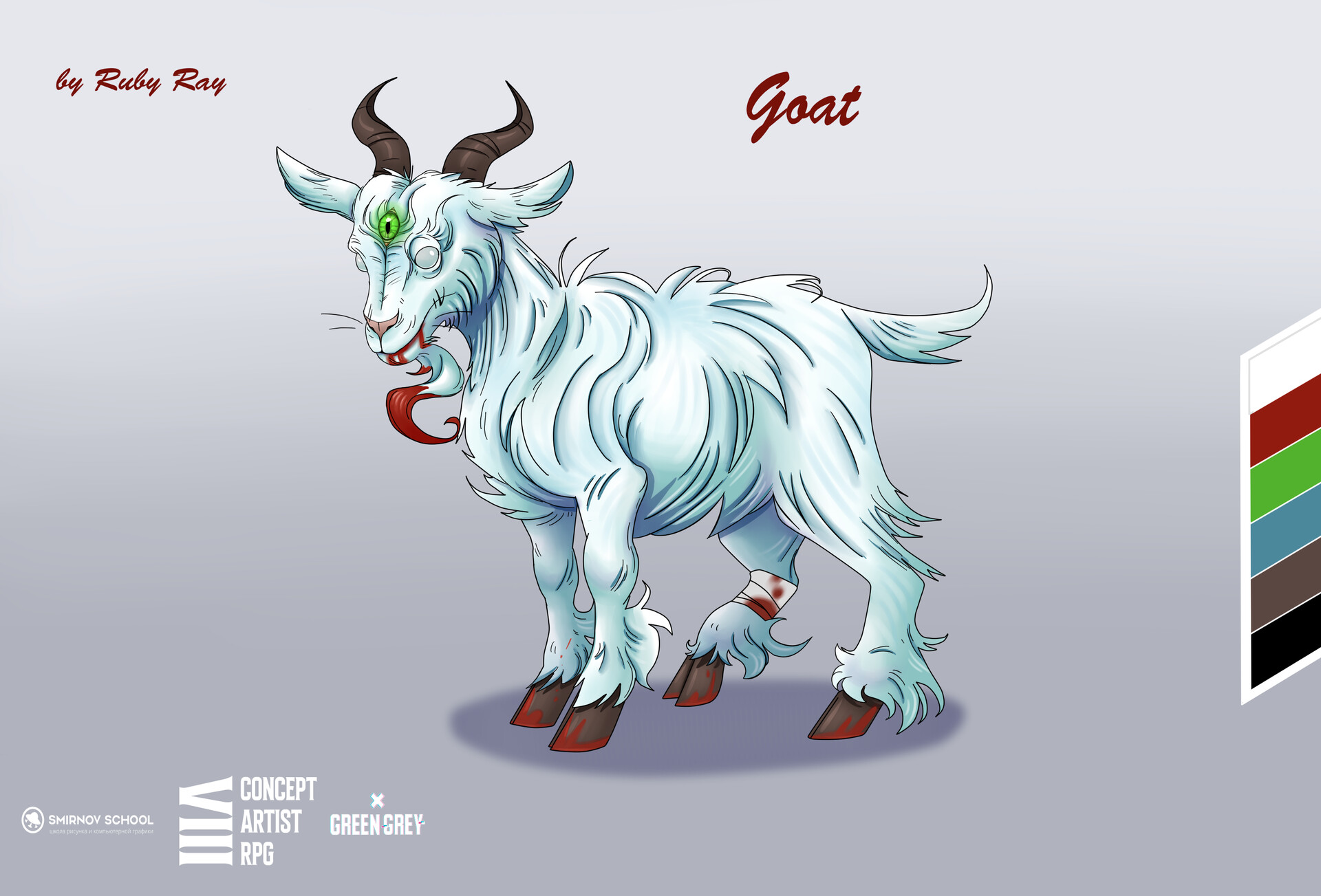This eerie illustration titled "Goat" showcases a mystical, demonic white goat with a blue tinge. The goat sports two brown horns, bloodstained hooves, and a small goatee similarly marked with blood. Blood drips from its mouth, adding to its menacing appearance. Uniquely, the goat has a third eye in the middle of its forehead that glows bright green, contrasting with its two white eyes. The goat stands on a silhouetted circle, and its right hind leg is wrapped in a blood-soaked bandage. The top center of the image displays the label "Goat" in red text, while the credit "by Ruby Ray" is in the top left-hand corner. The bottom left-hand corner bears a logo and the phrases "concept artist RPG X green gray." Additionally, a color palette featured on the right side of the image includes shades like white, red, green, blue, gray, brown, and black, highlighting the eerie and haunting tones used in the drawing.